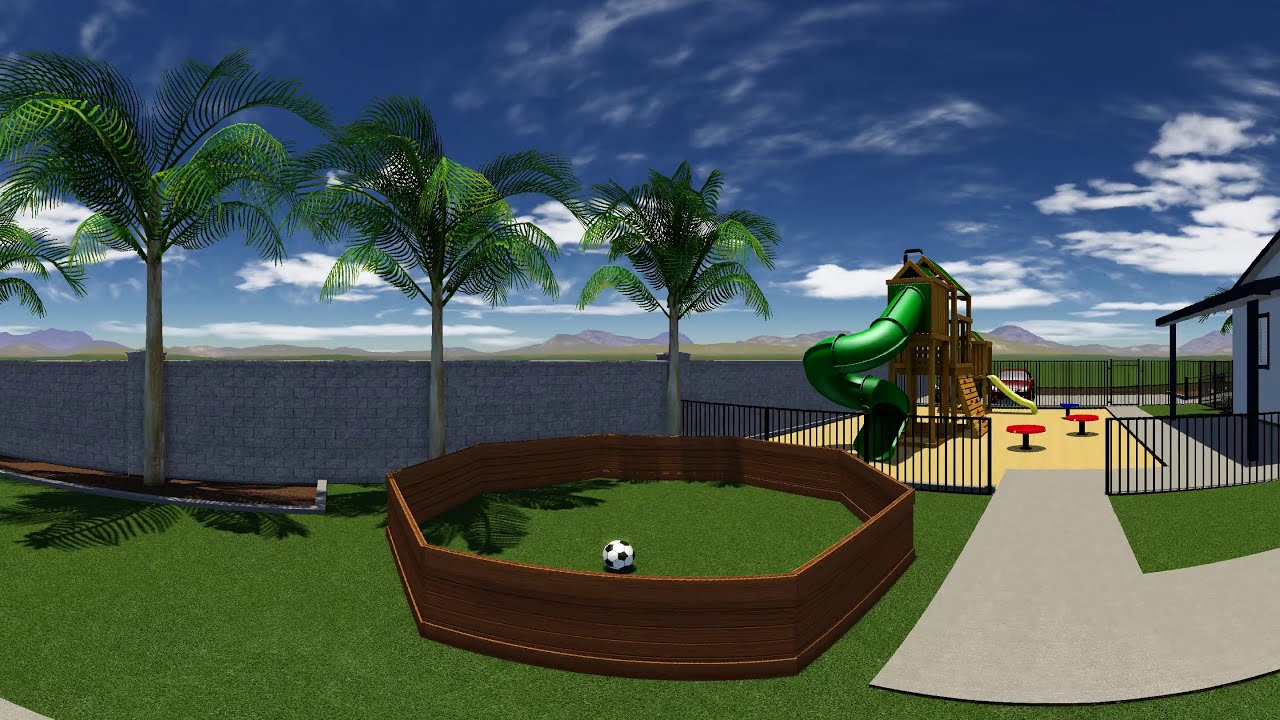The image depicts a detailed, computer-generated 3D outdoor scene centered around a playground near a house or school-like building. In the middle of the grassy area, there is a small wooden enclosure with a soccer ball inside. To the left of the enclosure stand three palm trees, and behind them, a gray fence runs along the scene's boundary. The playground, situated in front of the house on the right side of the image, features a large wooden climbing structure with a green tubular slide. Additionally, there are two small red benches nearby for seating. A paved sidewalk weaves through the grass, connecting the playground to the house, which appears white with brown accents and a black metal gate surrounding the playground area. The sky overhead is clear blue with white clouds, and in the distance, mountains can be seen, adding a sense of depth and natural beauty to the scene.